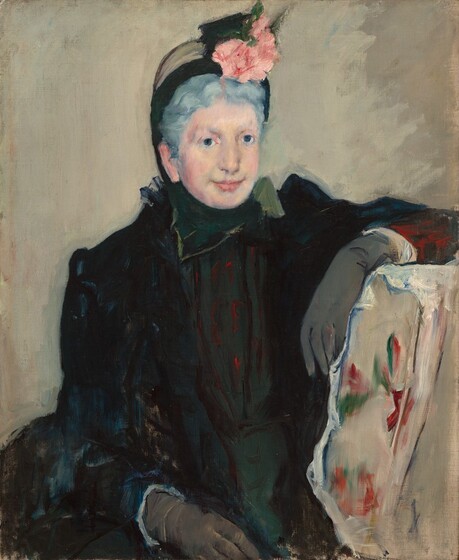This painting showcases an older woman with short gray hair, accentuated by her pale complexion, evident blush, and lipstick. She is adorned in very old-fashioned attire: a heavy black coat over a dark green dress which has subtle red vertical stripes. Her outfit is complemented by gray or dark brown gloves. 

The woman is slightly facing towards the right, with her left arm propped on the back of an ornate chair, and her right arm resting on her lap. The chair features a smushed floral pattern with predominately red flowers, green stems, a tan fabric, and what appears to be a white draping over it.

She wears a tan hood, and over it, a pink flower headdress sits prominently to the left above her eye. The background of the painting is also a soft tan, and the visible brush strokes indicate that it is likely an oil painting due to the way the colors blend together. The woman, who has a long nose, seems to be smiling slightly, adding a touch of warmth to the composition.